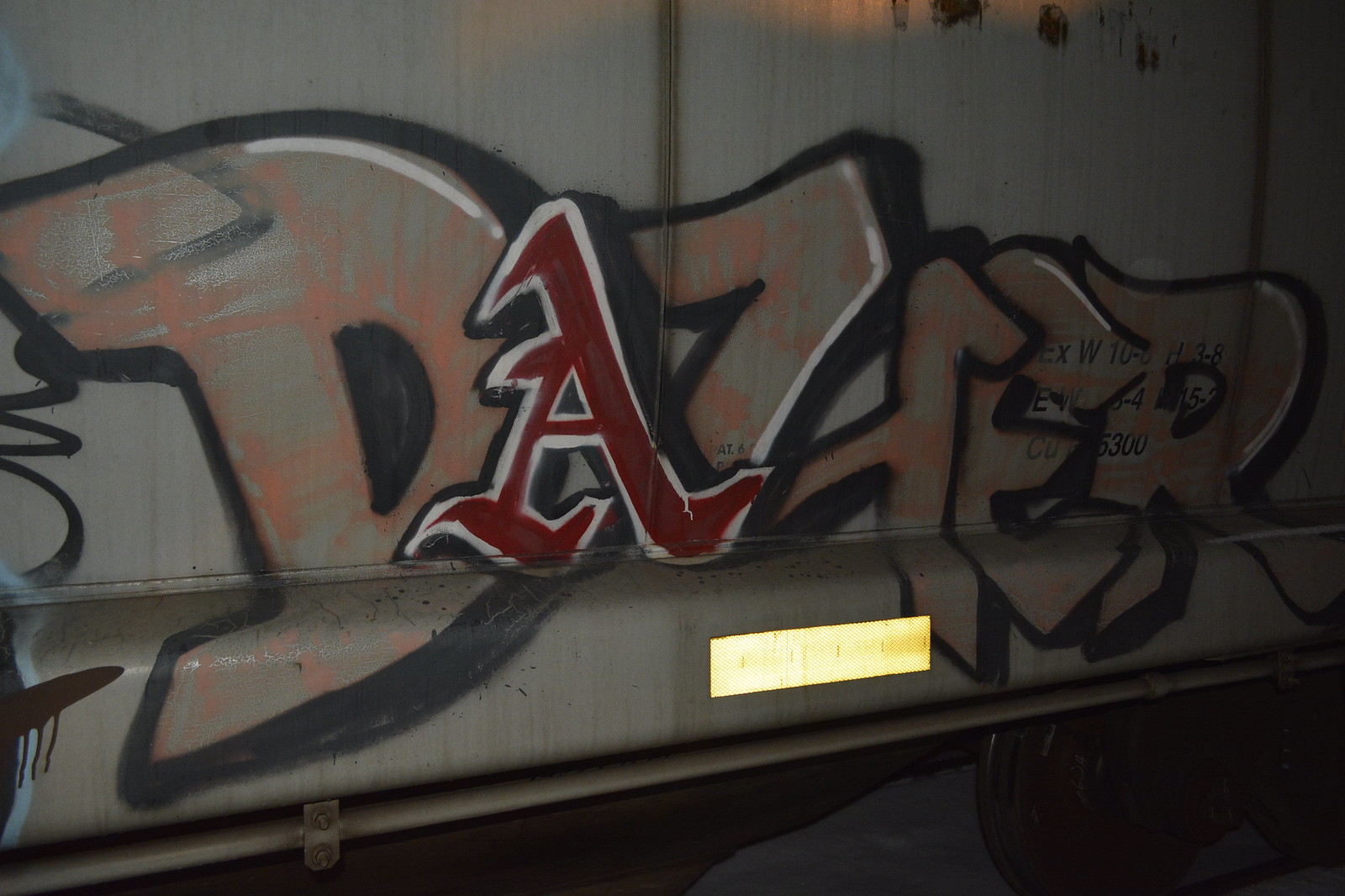The photo captures vibrant graffiti on the side of a train, prominently featuring the letters "D, A, Z, E, R." The letter "A" is distinctly stylized in red with a white and black outline, making it stand out strikingly. The letters "D, Z, E, R" are outlined in black with patches of peach color dispersed throughout, adding to the dynamic aesthetics of the art. Behind the letters "E" and "R," faintly visible are the characters "EXW," and the numbers "10" and "53." The lower part of the image reveals a train wheel, confirming the graffiti's placement on a rail car. Additionally, the scene includes a gold-colored rectangular plaque-like object, though its details are obscured by glare, and a bolted pipe further emphasizes the industrial context.